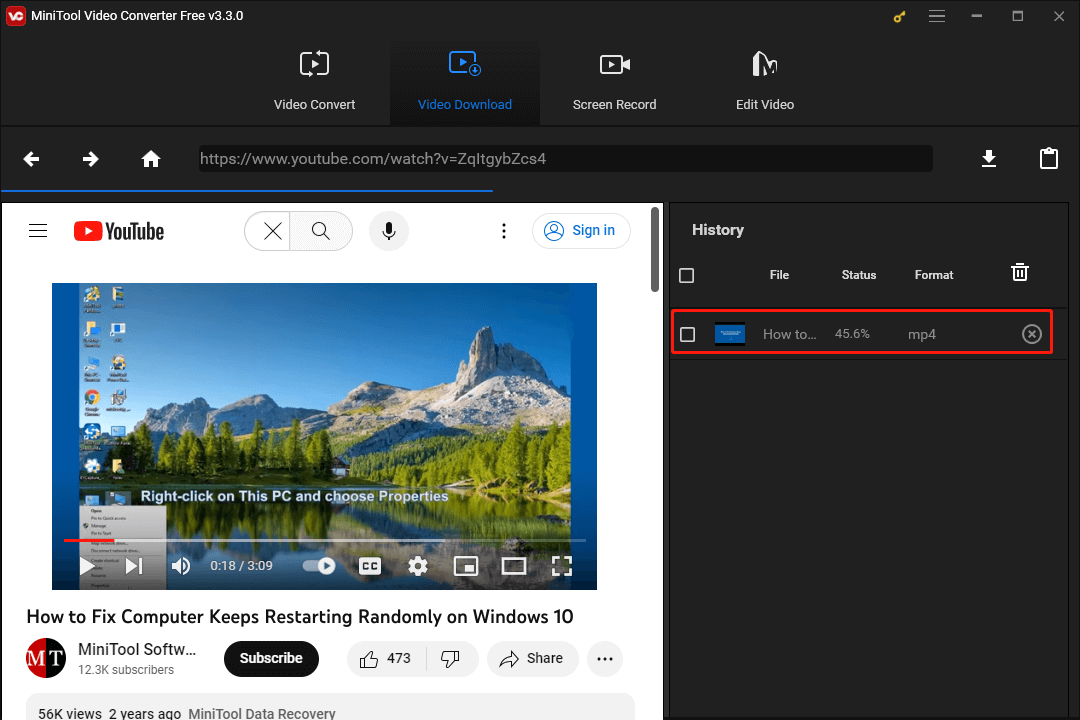This is a screenshot of a software interface, predominantly featuring a dark grey background. In the top left corner, there is a red square with rounded corners, displaying the text "WHITE VC" in all caps. Adjacent to it, in white text, reads "MiniTool Video Converter Free V3.3.0." On the far right, there is a clickable yellow key icon, followed by three horizontal lines, and the standard window control icons for minimizing, maximizing, and closing the screen.

Below this header, four options are displayed horizontally. The first option is "Video Convert," the second option, highlighted in blue, is "Video Download." The third option is "Screen Record," and the final option is "Edit Video." 

A web address is visible in a search bar below these options, indicating that the software is sourcing content from the internet. The URL is "YouTube.com/watch?v=ZQLTGYBZCS4."

The YouTube video currently open in the interface is titled "How to Fix Computer Keeps Restarting Randomly on Windows 10," and it has received 473 likes. The video's duration is 3 minutes and 9 seconds.